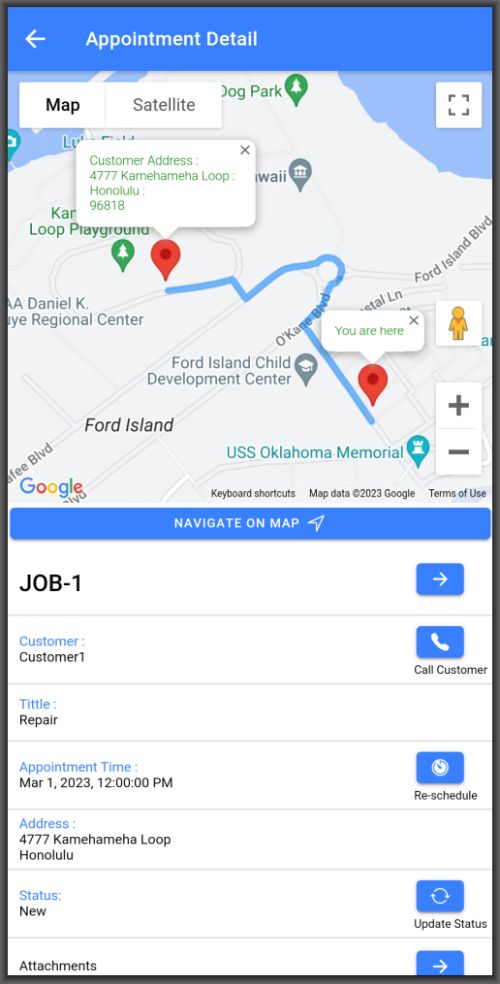The screenshot shows a smartphone display featuring a Google Map with a blue and black border. At the top, a blue banner contains a bright white left-facing arrow labeled "appointment deal." The map centers on the customer's address, "777 Kamaha Loop, Honolulu, 96818," and indicates "You are here" at the USS Oklahoma Memorial. A blue line connects the two locations.

Below the map is a navigation banner with a send icon. Further down, job details are provided: "Job-1" is labeled with a blue box and a white arrow. To the right is a blue square with a white phone icon labeled "Call Customer." The title "Repair Bill" is followed by an appointment time set for March 1st, 2023, at 12:00 PM, along with a blue box labeled "Reschedule."

Further details include the address "777 Kamaha Loop, Honolulu," with a status marked as "new." An "Update Status" button is displayed in a blue box, accompanied by an "Attachments" section, and to the right, another blue box with a white right-facing arrow.